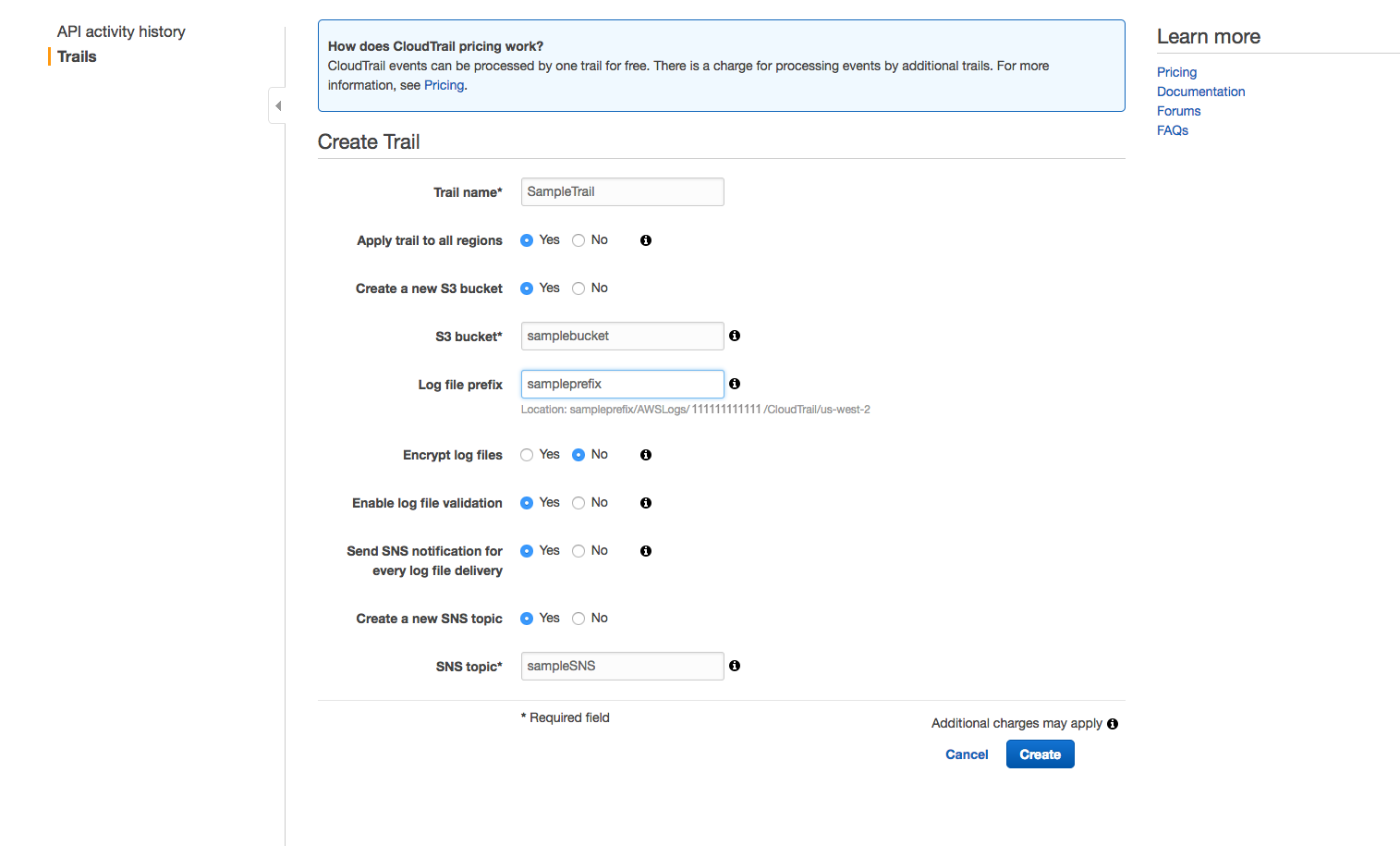**Caption:**

This image shows a screenshot of a settings page within the CloudTrail service. In the top left corner, the page title "API Activity History" is displayed, with the submenu item "Trails" listed directly below it. The "Trails" item is highlighted by a yellow bar to its left, indicating it is currently selected. Adjacent to this section, there is a button that appears to be a "Collapse" option.

The central section of the screenshot features a blue box at the top, with text explaining the pricing model for CloudTrail services: "How does CloudTrail pricing work?" This section notes that CloudTrail events can be processed by one trail for free, with additional charges applied for processing events by additional trails. A link labeled "Pricing" directs users to more detailed pricing information.

To the right of this text, there is a "Learn More" link, followed by a line separator. Below this, there are four buttons labeled "Pricing," "Documentation," "Forums," and "FAQs," offering quick access to pertinent resources.

Beneath the blue information box, in the middle section, is the "Create Trail" form. This form includes an empty field labeled "Trail Name" marked with an asterisk, indicating it is a required field. The placeholder text in this field reads "Sample Trail." Additionally, there is an option labeled "Apply Trail to All Regions" with corresponding "Yes," "No," and "Information" buttons available for selection.